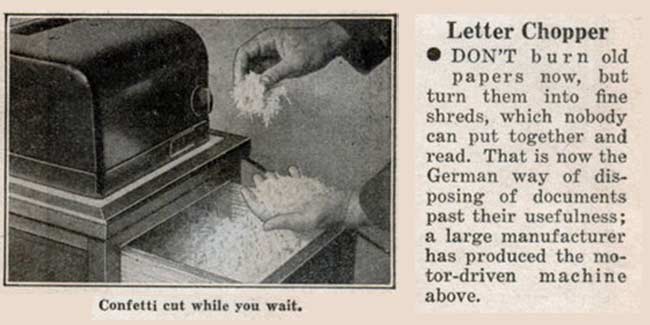The image is a black-and-white newspaper advertisement for an early model paper shredder, overlaid with a tan hue, possibly from age or digital editing. The photograph on the left side shows a paper shredder affixed atop a wooden cabinet. The shredder has a dome-shaped top with a visible dial and slot for paper insertion, somewhat resembling a toaster at first glance. The cabinet drawer is pulled out, revealing shredded paper, and a person, identified by their suit jacket cuffs, is holding a handful of the fine shreds in both hands. The image is bordered with a simple double-lined frame, consisting of a white line inside a darker, black line.

Below the photograph, the caption reads, "Confetti cut while you wait." To the right, the text prominently titled "Letter Chopper" advises, "Don't burn old papers now, but turn them into fine shreds which no one can put together and read. That is now the German way of disposing of documents past their usefulness. A large manufacturer has produced the motor-driven machine above."